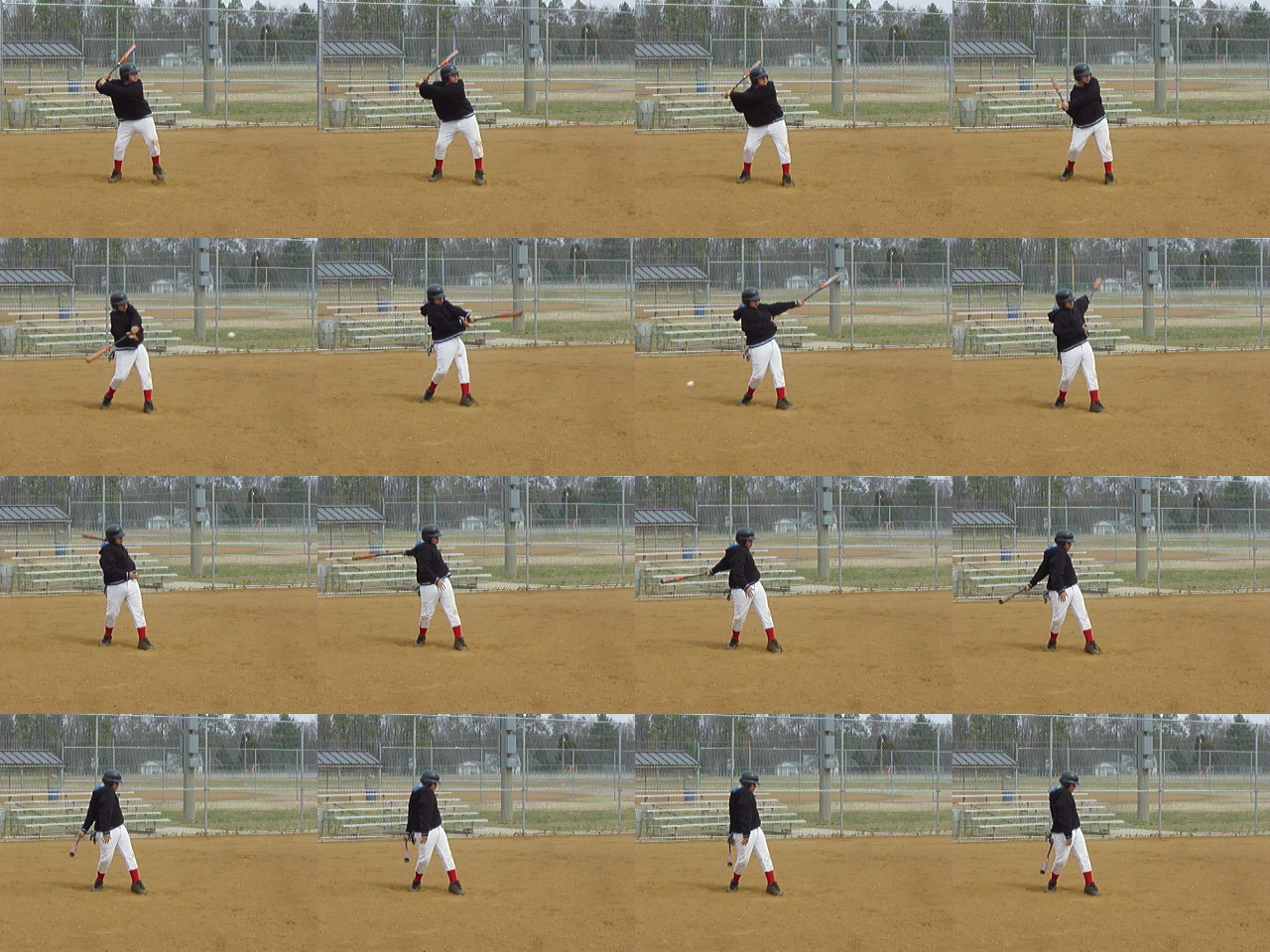This color photograph is composed of 16 smaller images arranged in a 4x4 grid, depicting a sequence of a baseball player at bat. The player, who is wearing a black helmet, black jersey, white pants, red socks, and black shoes, is pictured in various stages of preparing for and executing a swing. The sequence begins with the bat poised over his shoulders and progresses through the swing, showing detailed body movements as the bat comes down and then completes the follow-through.

In the background, there are empty bleachers, suggesting this takes place during practice rather than an actual game. Behind the player is a batting cage, and the setting includes green grass and distant trees. The ground in the foreground is a beige color, and there is a shadow cast from the right side, extending behind the player towards the left. The detailed progression of the swing across the images, with the ball's point of contact around the 7th image, and the player's final post-swing posture, suggests he may have missed the ball or hit a foul.